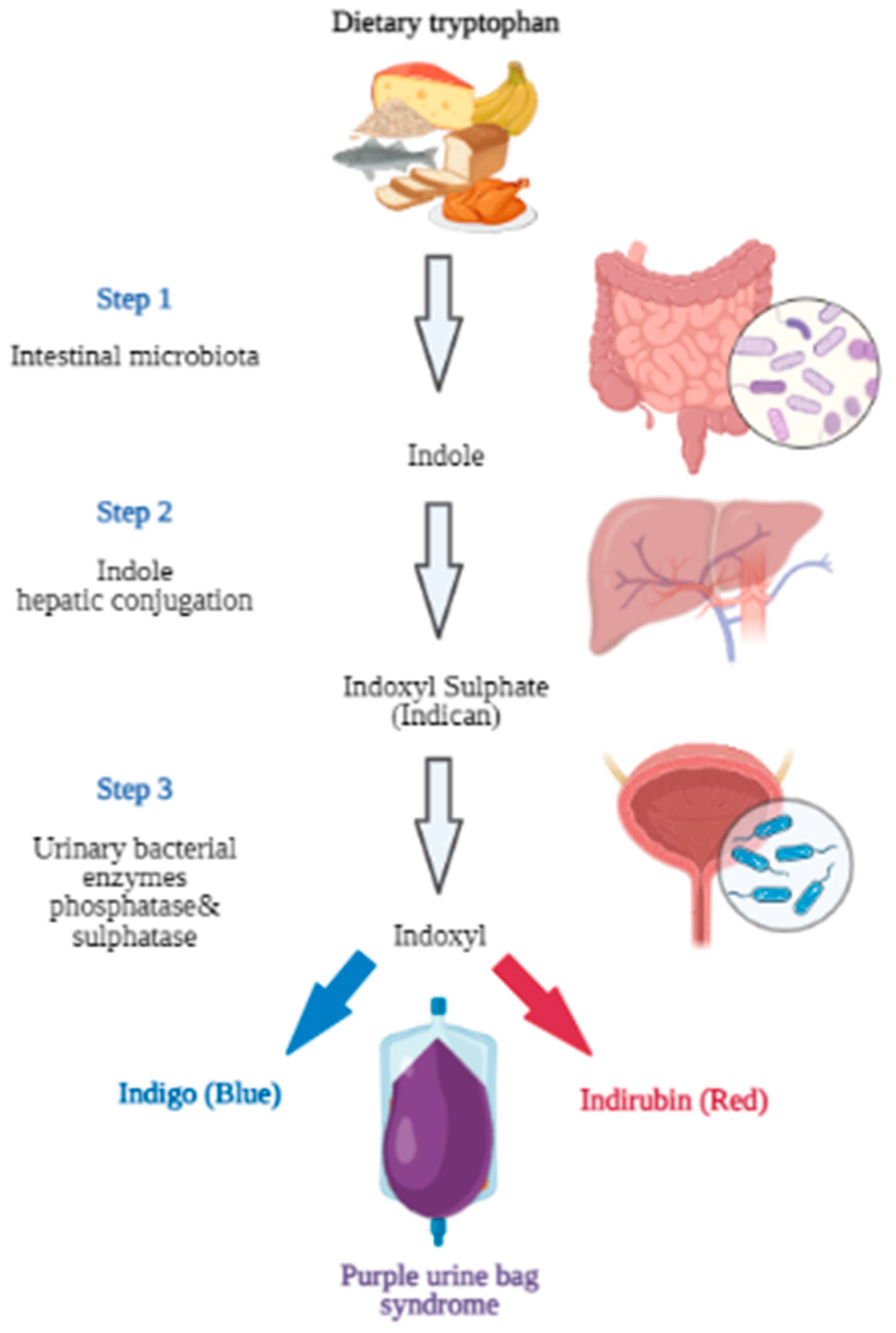The image depicts a detailed flow chart illustrating the biochemical process through which dietary tryptophan can lead to the condition known as purple urine bag syndrome. At the top, foods rich in dietary tryptophan—such as cheeses, bread, turkey, bananas, and fish—are illustrated, with an arrow pointing downwards. The first step highlights the role of intestinal microbiota in breaking down tryptophan into indole. This process is visually represented by the intestines on the right side. 

Next, indole undergoes hepatic conjugation in the liver, depicted in a subsequent step, transforming into indoxyl sulfate. The flow continues with indoxyl sulfate being further processed into indoxyl, which then splits into two pathways: one leading to indigo blue and the other to indirubin, marked in red. These color-coded transformations illustrate the chemical reactions responsible for the coloration.

Finally, urinary bacterial enzymes, specifically phosphatase and sulfatase—illustrated by the bladder—convert these compounds, ultimately resulting in the formation of purple indoxyl. The chart culminates with a visual of a urine bag containing a large, purple teardrop, labeled "purple urine bag syndrome," signifying the syndrome's characteristic symptom.